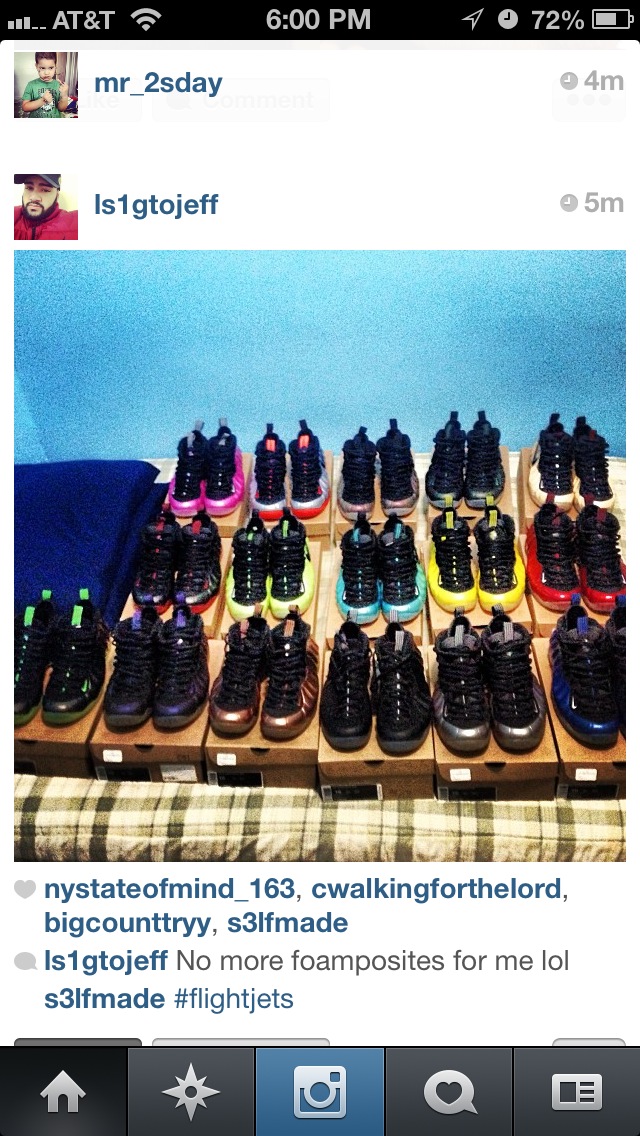An older screencap of an Instagram post taken on an iPhone using the AT&T network at precisely 6 p.m., with the battery level at 72%. The post, made by user is1gtojeff five minutes prior, features neatly stacked pairs of black sneakers, each set atop their respective boxes. The sneakers are identical in design but have varying sole colors—pink, silver, red, teal blue, yellow, green, purple, and black, indicating a diverse collection. At the top of the image, the carrier, time, and battery details are visible. The caption reads, "No more foam posites for me," with likes from several users including NYStateOfMine, WalkingForTheLord, BigCountry, and S3LFmade. The phone's menu bar is visible at the bottom, showing the Home, Navigation, Instagram, Like, and News buttons.